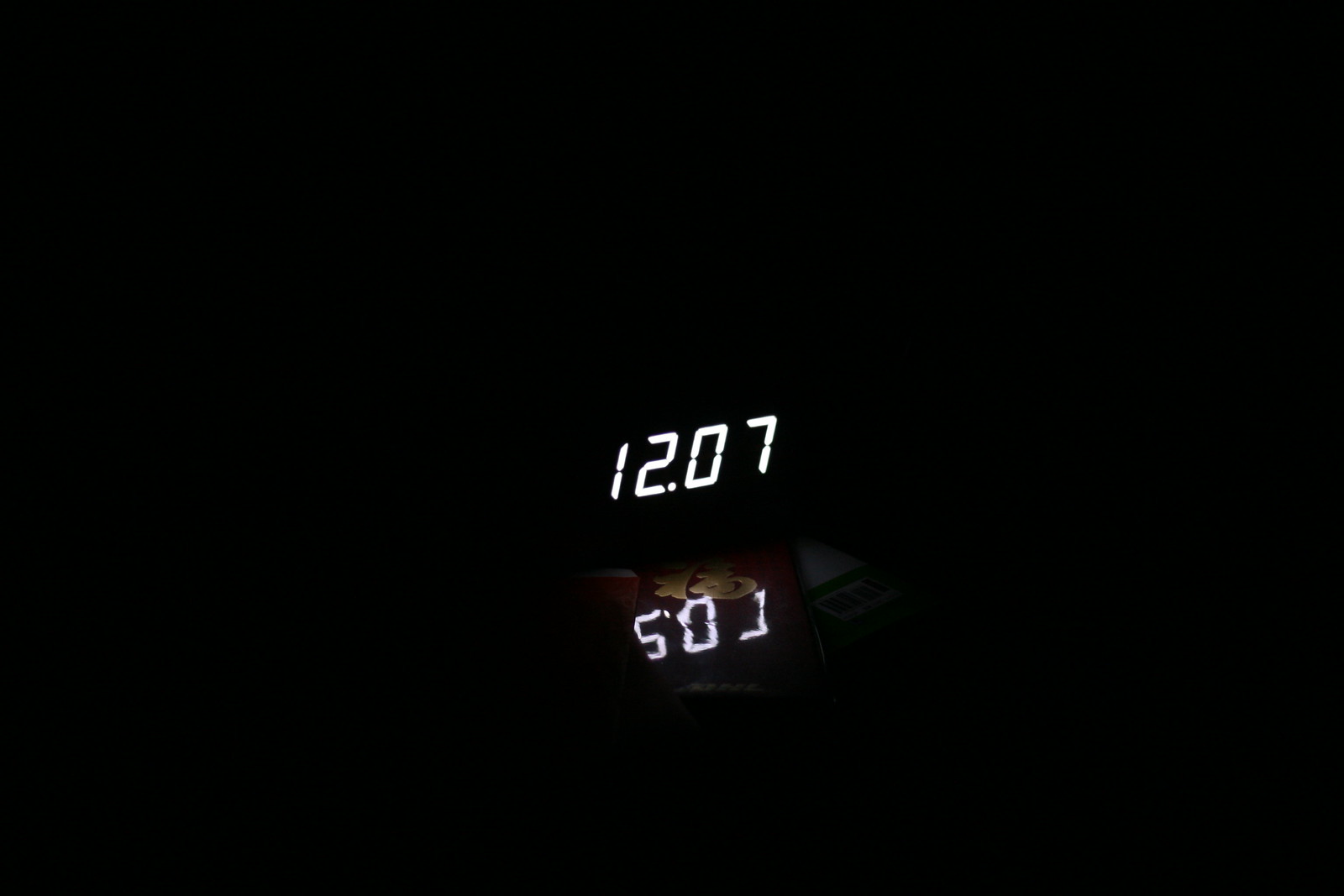In this image, a digital clock is captured in a dimly lit environment, resulting in most of the screen being shrouded in darkness. The luminescent digits of the clock stand out prominently, showing the time as "12.07" with a period separating the hours and minutes instead of the usual colon. The glowing display softly illuminates its surroundings, revealing the faint reflection of two objects. One appears to be an inverted book, identifiable by the visible green and white colors and a discernible barcode. The second object is more ambiguous but seems to be a red rectangle adorned with gold Asian or Chinese characters, adding an enigmatic cultural element to the scene.